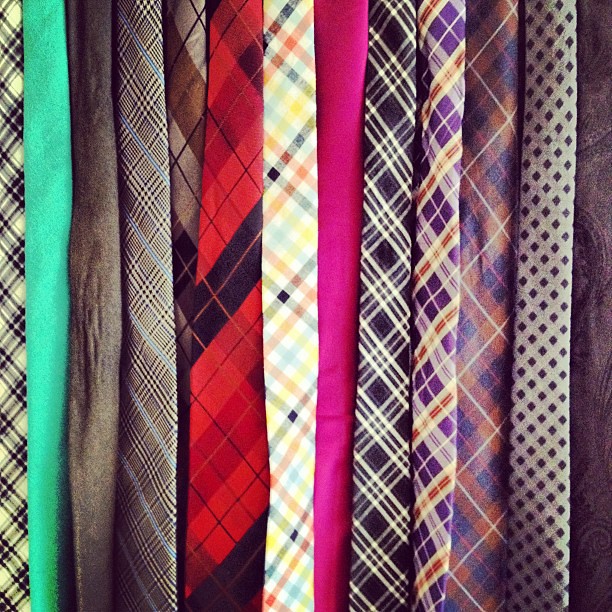This close-up photo captures approximately a dozen vibrant men's ties, arranged in neat vertical rows reminiscent of stripes. The image emphasizes the intricate and varied patterns of the ties, which include a black and white checked, a solid green, a solid gray, a gray and white checked, a brown checkered, and a red tartan pattern. There's also a multi-colored pattern resembling a tablecloth, a solid pink, a blue and white crisscrossed pattern, a purplish tie with brown highlights, a checkered bluish and brownish tie, a square pattern outlined in white, and a gray paisley design. The ties evoke a retro feel, possibly from the late 70s to 80s, suggested by their styles. The meticulously aligned ties, captured in a square, portrait-style orientation, create a curtain-like appearance, with only the hanging sections visible, showcasing their rich colors and complex designs in sharp focus.